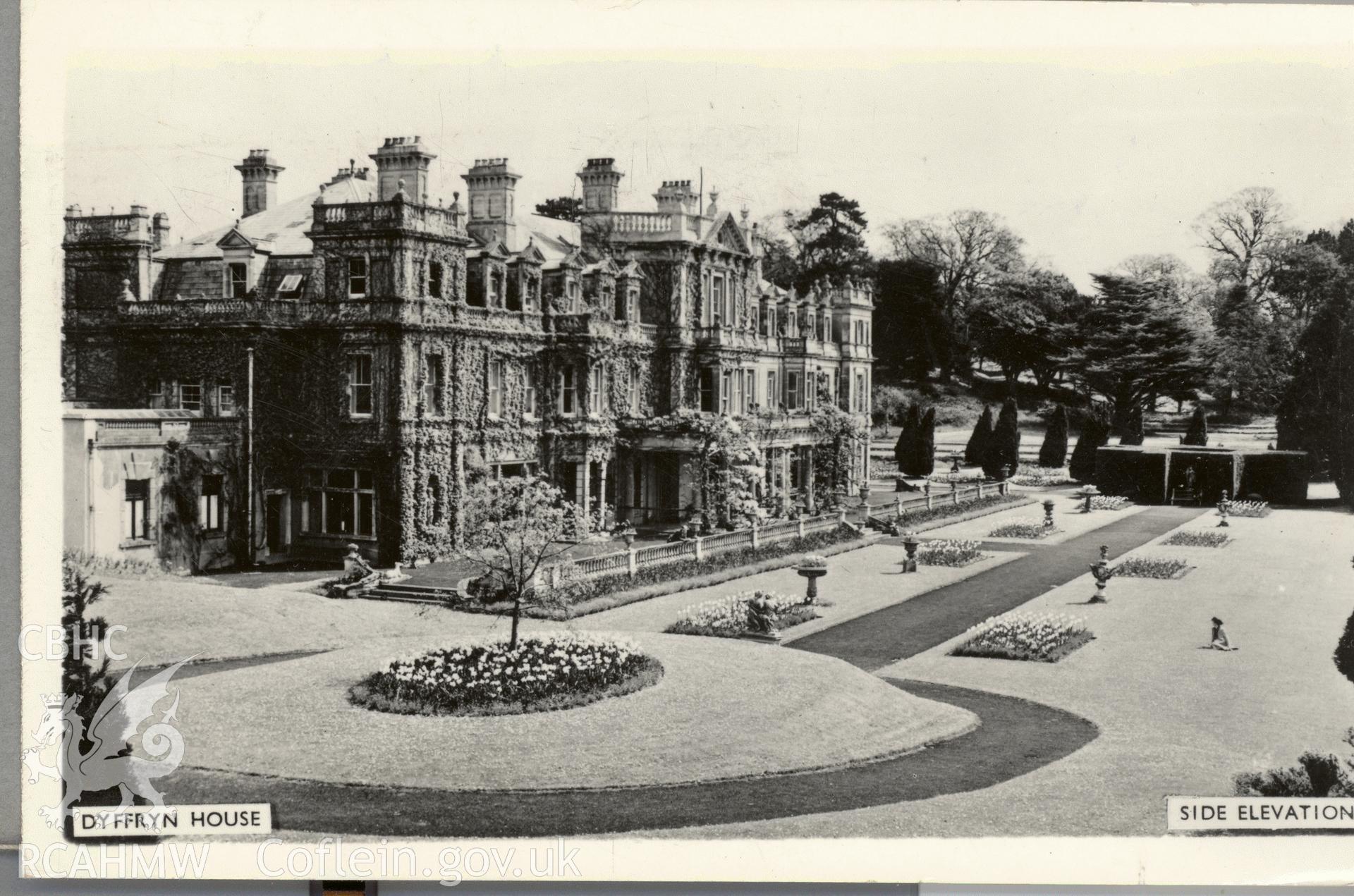This evocative black and white photograph, resembling a vintage postcard with visible print edges, captures the majestic grandeur of Dyffryn House. In the lower left corner, a white box with the text "D-Y-F-F-R-Y-N House" is seen, along with an emblem and the letters "CBHC" above it, framed with off-white and dark gray trim. On the lower right corner, a similar box is labeled "Side Elevation." The imposing three-story manor, adorned with numerous chimneys and flues, also features widow's walks and towers. Its elaborately decorated facade is partially veiled by vines and ivy, with a sprawling terrace across the front.

The meticulously landscaped gardens in the foreground showcase circular flower beds, manicured trees, garden statues, and a birdbath. A paved walkway circles a small hill adorned with a tree surrounded by flowers, continuing on to create an inviting garden path. Steps lead up to the main building from a grand sidewalk, while a young child can be seen sitting and enjoying the manicured grassy area to the right. The image also captures more gardens and a fence bordering the scene, enhancing the sense of a well-kept estate. In the background, a mix of evergreen and deciduous trees paint a serene natural backdrop, completing the stately and tranquil ambiance of this historical residence.